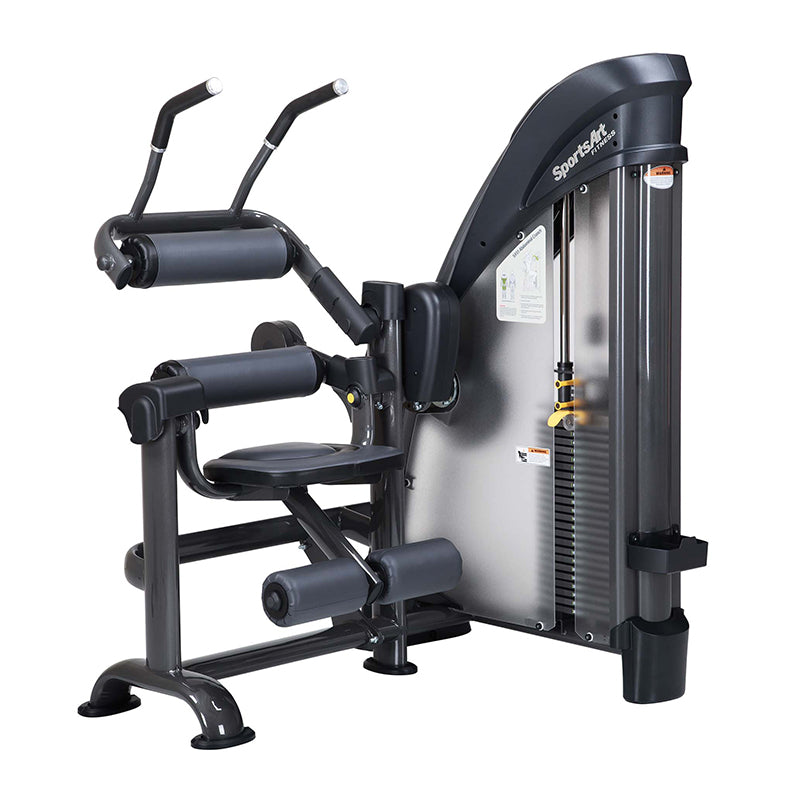The image depicts a piece of sophisticated workout equipment branded Sports Art Fitness, primarily in dark gray and black colors. It features a detailed and multi-functional design tailored for abdominal exercises. Positioned on the right side of the machine, the Sports Act logo is prominently visible just above a weight selection mechanism. Users can set their desired resistance level here, indicating it's customizable for different fitness levels.

On the left side, the equipment is equipped with three different padded cushions. At the top, there are handlebars situated near a cushion, likely for arm support during exercises. Below this, there's a cushioned seat with an accompanying backrest, designed for comfortable seating. Further down, a footrest area is also cushioned, ensuring stability and comfort for the user's feet.

Visible beneath the Sports Act logo are weights integrated within the machine, with their setting adjustable through an adjacent small diagram. The foot area and pedals, along with handles, appear to be strategically placed for engaging in various workout motions, enabling the user to perform movements like leg lifts or crunches while pulling down on the handles to work the abdominal muscles. The equipment exudes a solid, grounded structure, ensuring stability during intensive workouts.